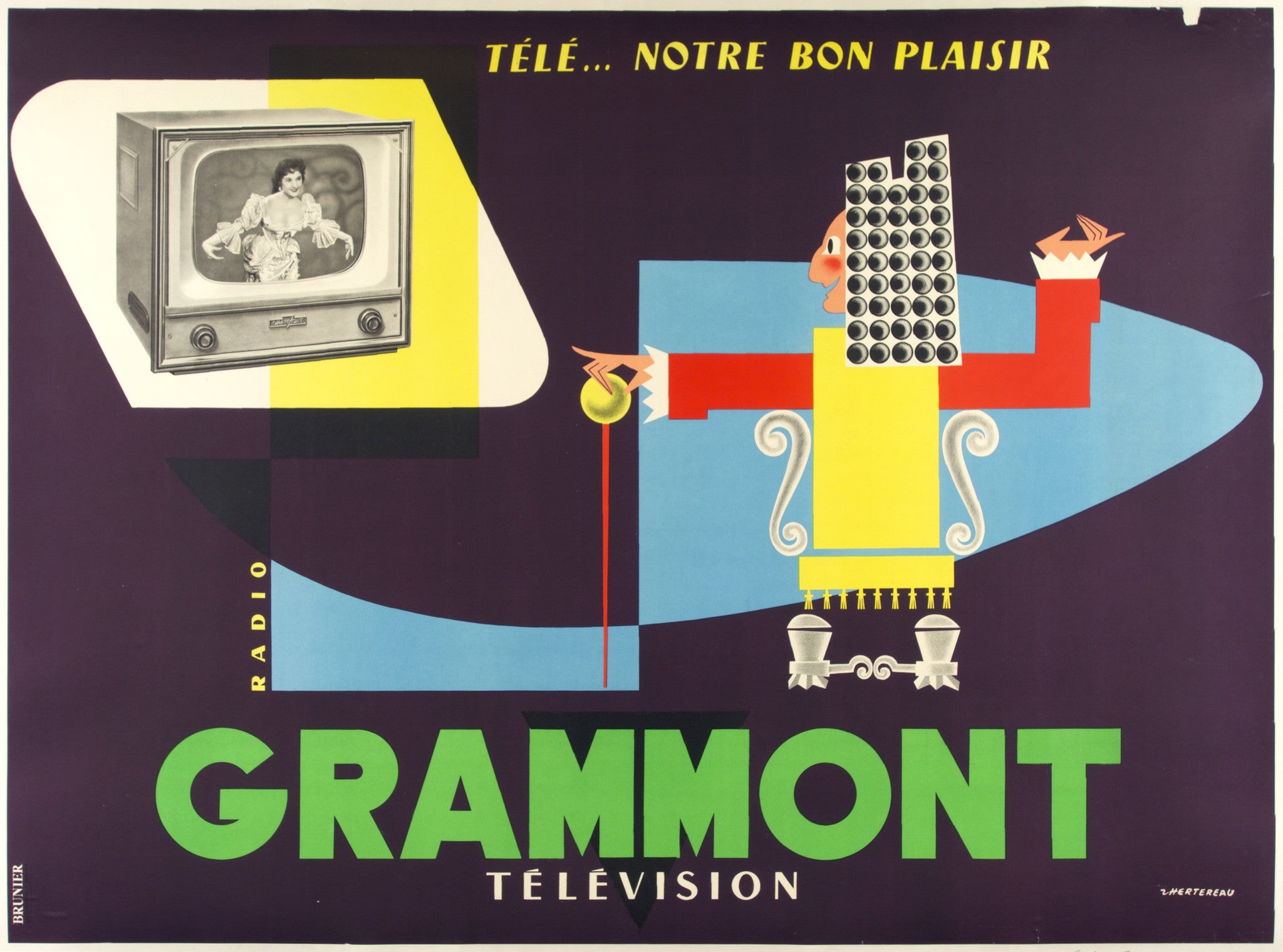This image, likely an advertisement for a television streaming platform, showcases a vibrant, old-school animated aesthetic. At the top, French text reads "Télé... notre bon plaisir," which translates to "Television, our good pleasure." The dark, nearly black background accentuates the colorful elements. Positioned in the top left corner, a vintage black-and-white CRT television displays a woman in an elaborate dress, bowing. To the right stands a cubist-style animated figure, possibly resembling a French king, adorned in a yellow tunic with red sleeves and white lace cuffs, and iconic, stylized hair. Blue accents and vertical yellow text spelling "RADIO" further enhance the retro look. At the bottom center, "Grumont Television" is prominently displayed in large green and white text, likely indicating the producing studio behind this classic-themed advertisement.